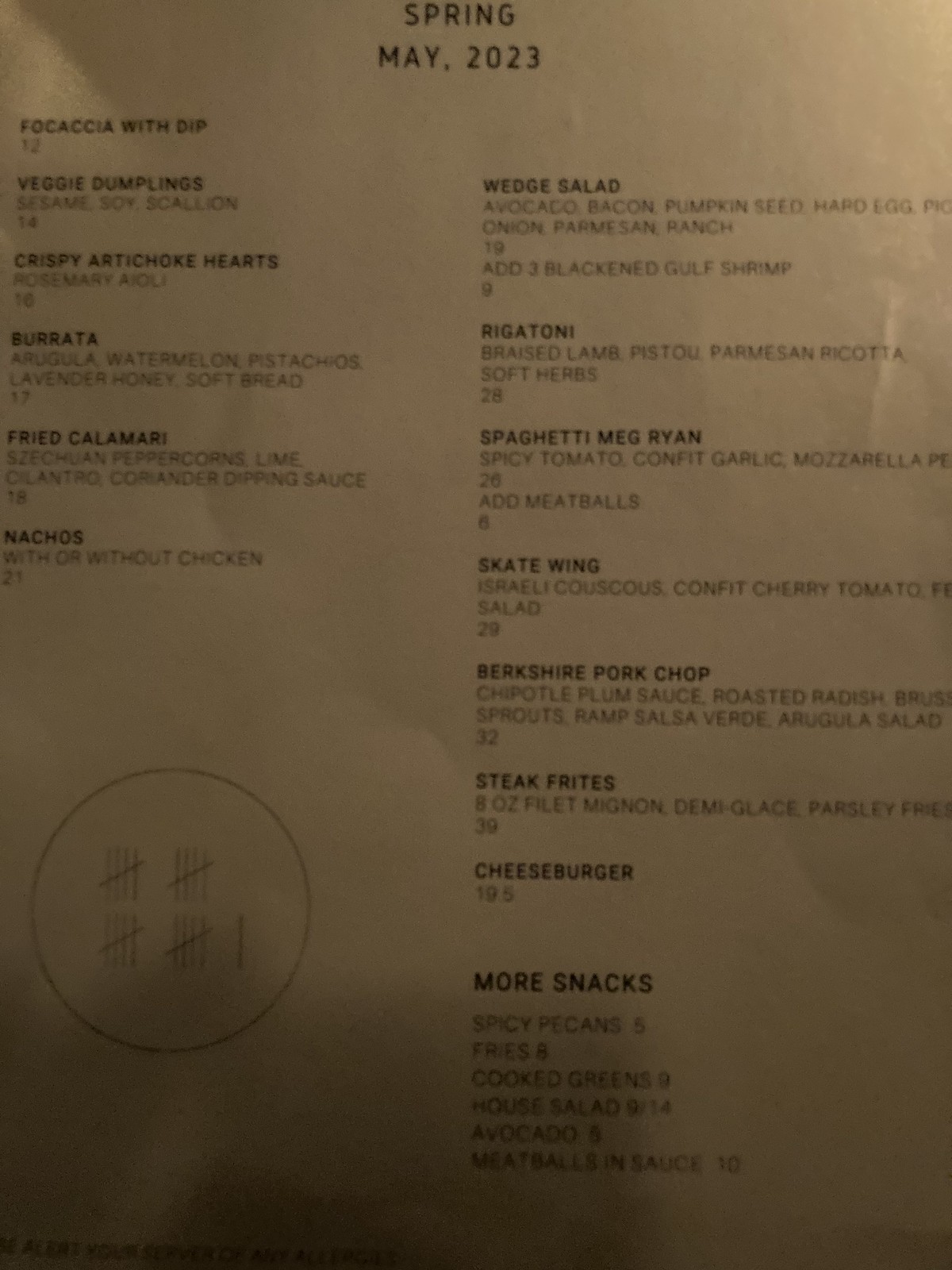This image captures a dark, portrait-oriented menu printed on light brown paper. The menu details various dishes available during Spring, May 2023. 

In the left column, the menu lists:
- Focaccia with Dip - $12
- Veggie Dumplings with sesame, soy, and scallion - $14
- Crispy Artichoke Hearts with rosemary aioli - $16
- Burrata with arugula, watermelon, pistachios, lavender honey, and soft bread - $17
- Fried Calamari with sushi peppercorns, lime, cilantro, coriander, and dipping sauce - $18
- Nachos (with or without chicken) - $23

On the upper right corner, the second column includes:
- Wedge Salad with avocado, bacon, pumpkin seed, hard-boiled egg, onion, and Parmesan ranch - $19, with an option to add three blackened Gulf shrimp for an additional $9
- Rigatoni with braised lamb, pesto, Parmesan ricotta, and soft herbs - $28
- Spaghetti 'Meg Ryan' with spicy tomato, confit garlic, and mozzarella - $26, with an option to add meatballs for an additional $6
- Skate Wing with Israeli couscous, confit cherry tomato salad - $29
- Berkshire Pork with chipotle plum sauce, roasted radish, sprouts, ramp salsa verde, and arugula salad - $32
- Steak Frites with filet mignon and demi-glace - $39
- Cheeseburger - $19.5

In the snacks section, the menu offers:
- Spicy Pecans - $5
- Fries - $8
- Cooked Greens - $9
- House Salad - $9
- Avocado-based dish - no specified price
- Meatballs in Sauce - $10

The overall impression suggests that the menu items are on the pricier side.